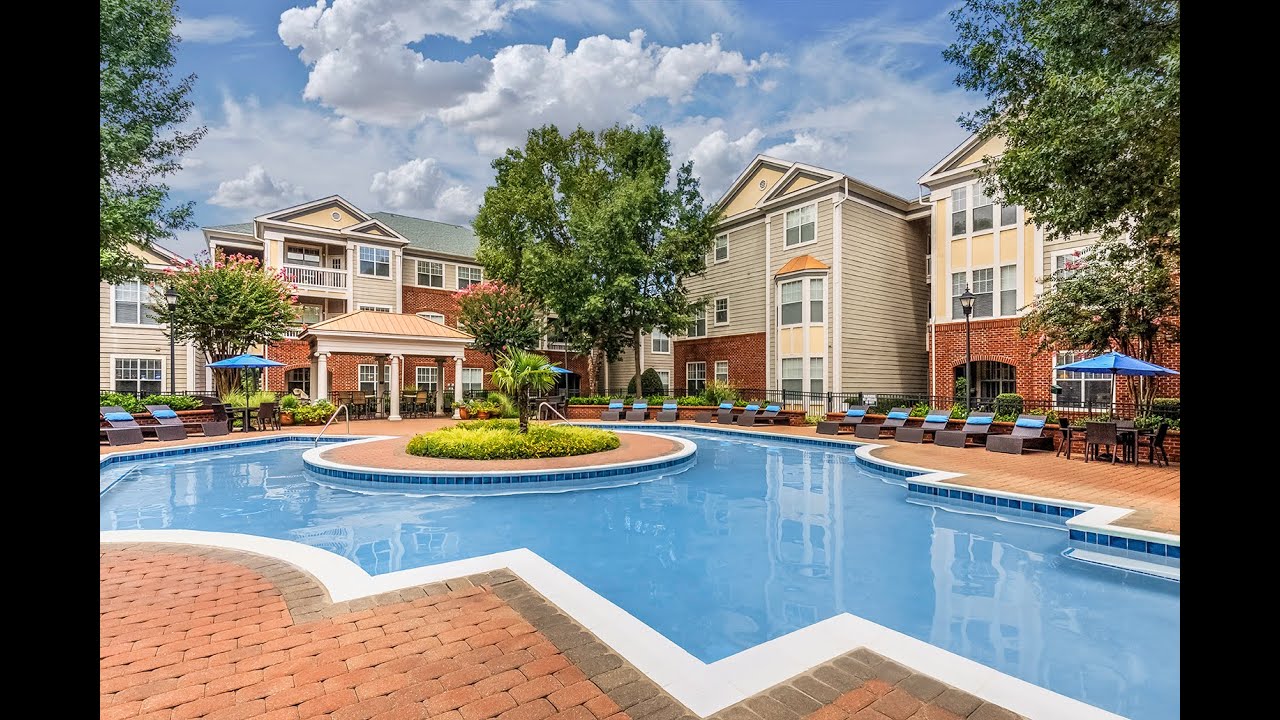This image is a detailed computer-aided conceptual rendering of a modern residential complex, likely comprised of apartment buildings or townhomes. Each building, which stands three stories tall, features tan siding with brick bases. Several of these buildings intersect at a 90-degree angle, creating a cohesive community layout. 

At the center of the image is a bright blue outdoor swimming pool, surrounded by a red brick patio area lined with a gray brick border. The pool includes a circular island adorned with green shrubs and a small palm tree. Adjacent to the pool, there are various lounge areas strewn with black lounge chairs that have blue pillows, and tables with blue umbrellas, which suggest a comfortable, leisurely environment. Surrounding the pool are tall, overhanging trees positioned to the right, left, and center of the image.

The sky overhead is depicted as bright and light blue with fluffy white clouds, enhancing the serene, resort-like atmosphere of the scene. The complex is designed to evoke feelings of luxury and relaxation, akin to a hotel or a resort setting, complete with a small pavilion in the background adding to the communal ambiance.